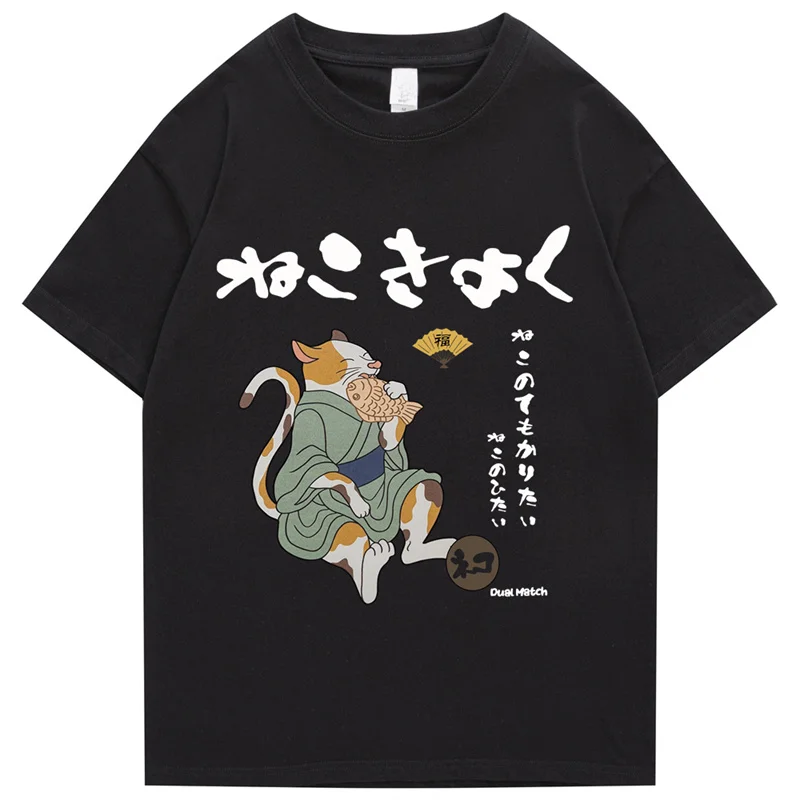This image features a unique black t-shirt displayed against a plain white background, possibly as part of a product mock-up. Dominating the design at the top, large white Asian characters, likely Japanese, span across the shirt, accompanied by two vertical columns of additional characters on the right side. The rightmost column is notably taller, twice the height of the adjacent column. Just off-center to the right is a traditional yellow paper fan with a dark brown handle. Below the columns of text is a dark brown circle containing black letters. Toward the bottom right of the shirt, there are white English words that appear to say "dual match." The focal point of the design is a detailed, cartoon-like depiction of a calico cat with white, orange, and brown patches. The cat is dressed in a light olive-green robe, tied with a medium military blue belt, and is shown sitting with one leg stretched out and the other bent, its tail curled behind it. The cat's eyes are closed as it munches on a fish, exuding a whimsical and serene aura.